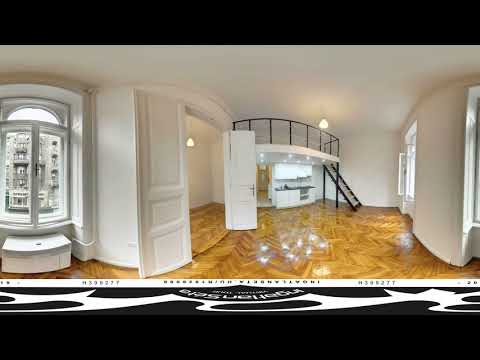The image depicts a bright, modern interior room with all-white walls and a ceiling. The floor consists of glossy, golden patterned parquet wood. On the left side, a large, tall rectangular window with a half-moon top is framed by white ledges and wainscoting. A small white chest sits in front of the window sill. To the right of the window, a white-plastered entryway leads to either another room or a closet, featuring the same flooring and a single pendant light hanging from the ceiling. 

Further to the right, the room opens into a kitchen with white cabinets and dark countertops. Adjacent to the kitchen, a hallway extends into the distance, while on the far right, a staircase with black and white treads ascends to a loft area. This loft, overlooking the kitchen, sports a black wrought iron railing. The room contains a wall with more large white windows on the right. At the bottom of the image, there is a black background logo with white text, possibly indicating a real estate advertisement. Overall, the space is minimalistic yet elegant, bathed in natural light, and designed for a harmonious, airy ambiance.